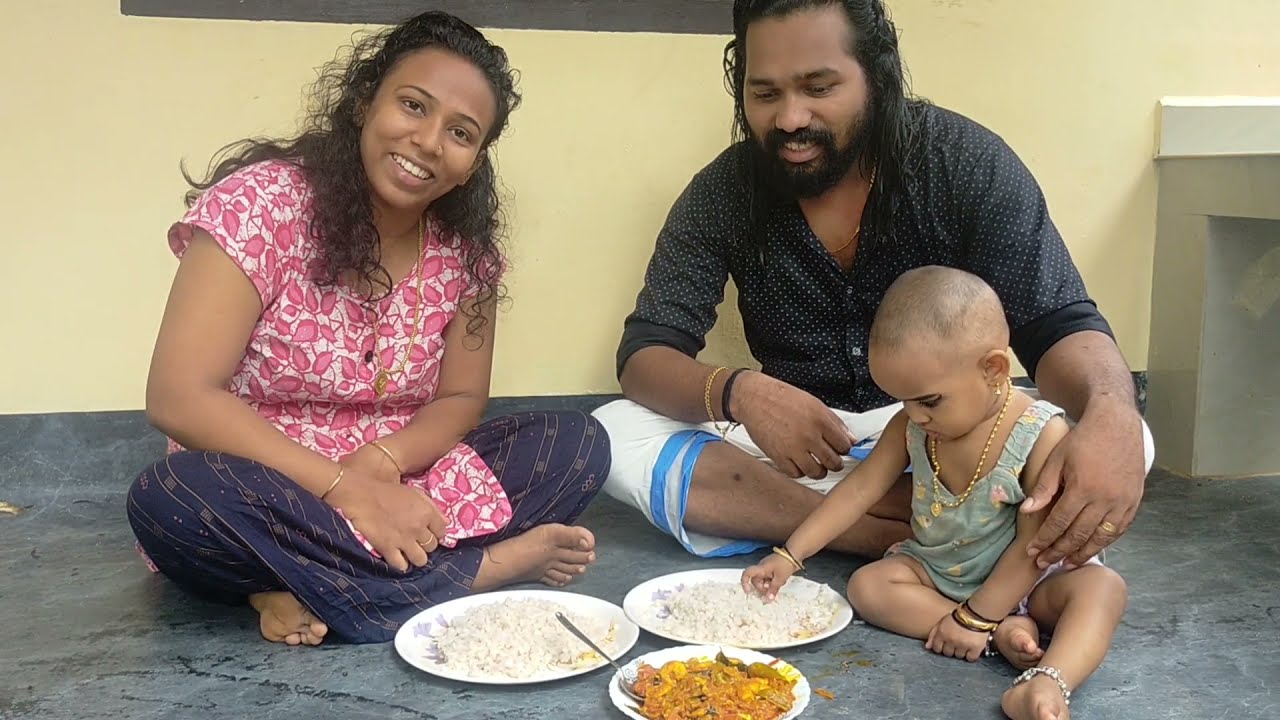This color photograph captures a presumably young family of three sitting barefoot on a black and gray marbled floor inside a home, adjacent to a pastel yellow wall. On the left is a smiling woman with dark curly hair cascading below her shoulders. She is dressed in a pink and white floral short-sleeve blouse paired with dark blue pants embellished with a gold pattern. To her right is a man with long wavy hair, a beard, and a mustache, clad in a dark navy or black patterned button-up shirt and white shorts with blue trim. He gazes downward at a small round plate of what appears to be an orange and yellow-colored dish positioned in front of him. Next to him sits a young toddler, possibly a girl, adorned with a gold necklace, bracelet, and earrings, dressed in a colorful romper. The toddler reaches towards another white plate of rice situated in front of them. Additionally, there are two more plates of food: one in front of the woman and another between the couple and the child, containing a yellowish dish with a metal spoon. In the background, part of a brown rectangle, possibly the frame of a photograph or mirror, is partially visible at the top of the image.